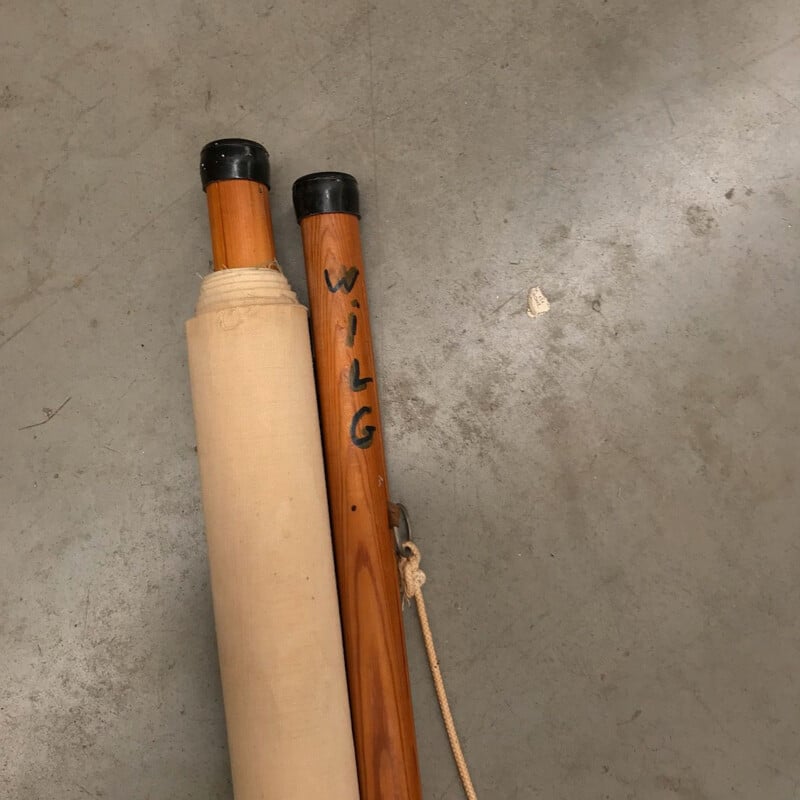The photograph showcases two wooden dowels with black plastic caps on both ends, lying parallel on a gray concrete floor. The dowel on the left is primarily wrapped in a canvas or parchment-like material, suggesting it is either a map or a display element. The right dowel remains mostly uncovered, featuring the letters "W-I-L-G" written vertically in black marker near its top. About six to eight inches down from the top of this dowel, a metal eye loop is attached, through which a white string is threaded and securely tied, likely intended for mounting the apparatus on a wall. The entire setup is positioned centrally and slightly towards the bottom of the frame, with a streak of light subtly illuminating part of the scene.